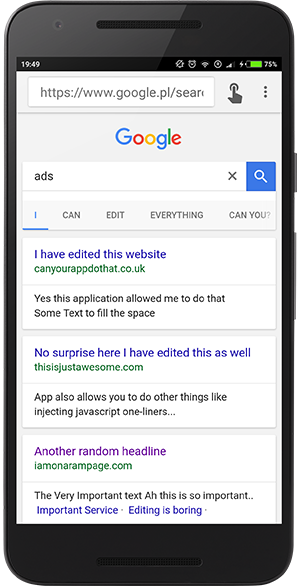In the image, a black iPhone displays a Google search results page. The status bar at the top shows the time as 19:49, alongside icons for signal strength and a battery level at 75%. Below this, the URL box displays "www.google.pl/search," accompanied by a finger icon and three vertical dots indicating a menu for additional options. Centered on the screen is the Google logo, with the search term "ads" entered in the search box.

The initial search results feature three visible links:
1. "I have edited this website. Can your app do that? - co.uk"
2. "No surprise here, I have edited this as well. - thisisjustawesome.com"
3. "I am on a rampage - onarampage.com"

The iPhone’s physical details include a speaker at both the top and bottom, emphasizing its black coloration. A finger appears to be pointing towards the screen, possibly interacting with the search interface.